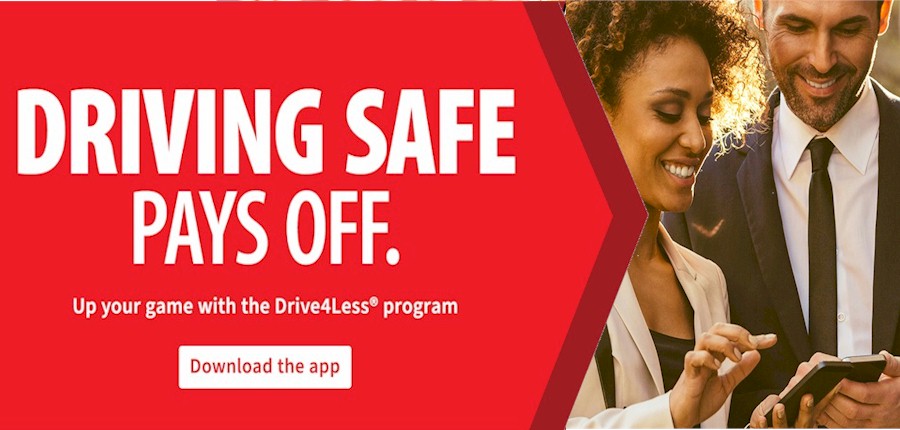A detailed banner features a horizontally elongated rectangle with a dominant left section in bright red, tapering to a point past the center. This red section includes a darker red stripe at the pointed edge adorned with large, bold, white capital letters reading "DRIVE SAFE." Below, in slightly smaller but still prominent white capital letters, the message continues with "Driving Safe" at the top and "Pays Off" beneath, followed by a period. Underneath in smaller font, it says "Up your game with the Drive for Less program."

Below this text, there is a white button with red text that says "Download the App."

On the right side of the banner, occupying the lower right corner, are two people—a man and a woman—both dressed in business attire. The man wears a white shirt with a brown tie and jacket, has a mustache and beard, and holds a black cell phone while smiling. The woman has a tan jacket over a brown shirt, with loose curly hair, and also smiles while looking at her black cell phone. She is black, and he is white. Their hands appear slightly crowded in the composition, suggesting a touch of AI enhancement. The overall scene conveys a positive and professional atmosphere, emphasizing the importance of safe driving.